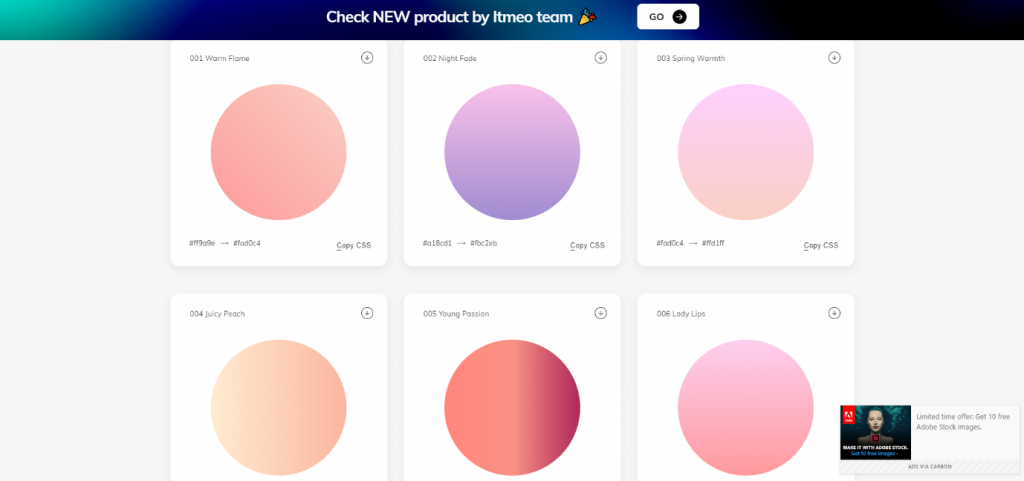This detailed caption would offer a clear and vivid description of the image:

The image, captured in landscape mode, appears to be a screenshot taken from a laptop screen. The top row features a gradient selection of colors beginning from light green, transitioning to teal, dark blue, and blue, culminating in black at the upper right corner. At the upper center of the screenshot, it reads "Check new product by ITMEO team," accompanied by an icon resembling a cornucopia. Below this text, there is a white button labeled "Go."

Beneath this section are two rows, each containing three images. These images are color swatches set against a white background, contrasting with the gray background of the remaining area. Each swatch includes a circular color sample and a label in the upper left corner, though the text appears blurry.

In detail:
- The first swatch in the top-left shows a coral color, labeled "001 Warm Flame." Numbers are listed below, and the bottom right of the swatch reads "Copy CSS."
- The second swatch is violet, labeled "002 Night Fade."
- The third swatch displays a light pink color, labeled "003 Spring Warmth."

Each of these swatches features a gradient that transitions from a darker shade to a lighter one.

In the bottom row:
- The first swatch displays a shade named "Juicy Peach."
- The second is labeled "Young Passion."
- The third features the color "Lady Lips."

At the bottom right corner of the image, there is a promotional message stating, "Limited time offer: Get 10 free Adobe Stock images."